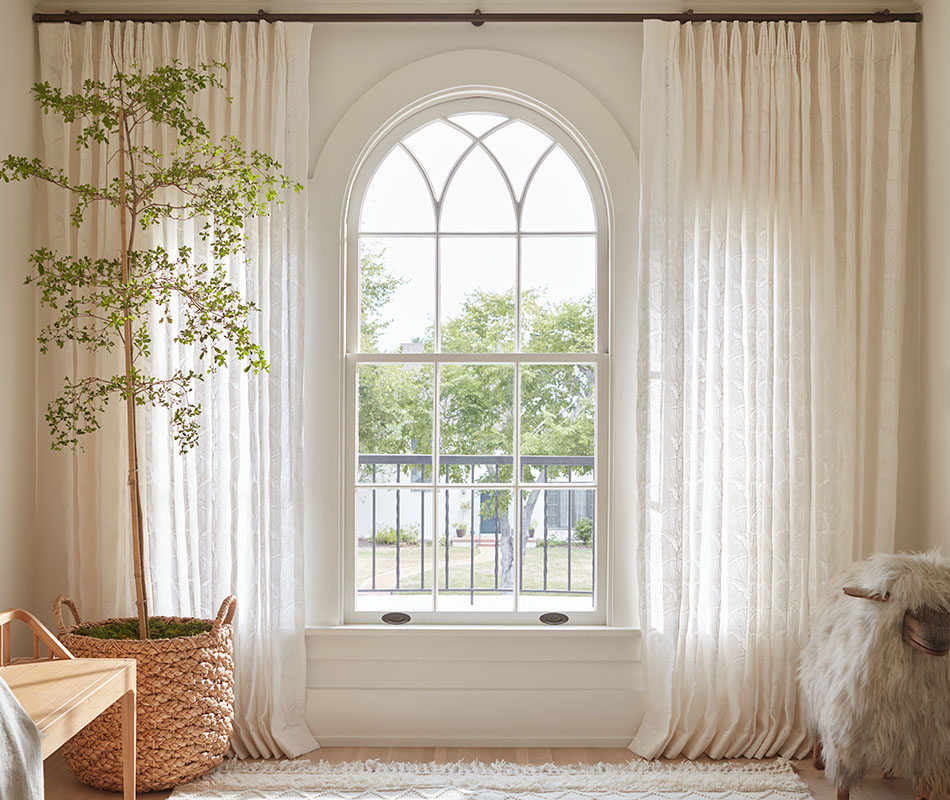This photograph captures a cozy and elegant room inside a home, focusing on a large, dome-shaped window with ornate panels. The black curtain rod at the top, bolted to the walls, supports white sheer curtains drawn open to reveal the view outside. The window, almost extending from the ceiling to just inches above the floor, floods the room with natural light. 

Through the window, you can see a home across the street, framed by a yard with trees, a fence, and potted plants. Inside the room, the flooring is light wood, adding to the airy ambiance. To the left, there's a tan wicker basket holding a small tree with sparse, tiny green leaves, which reaches from floor to ceiling. Partially obstructing the view of the tree, a piece of cloth drapes over the arm of a nearby chair. 

On the floor, a white frilly rug adds a touch of softness, accompanied by a light tan colored bench. On the right side of the room, there is a child's ride-on toy, resembling a furry sheep with a little black face, standing on wooden legs. The overall atmosphere of the room is serene and beautifully structured, with elegant details and charming elements throughout.